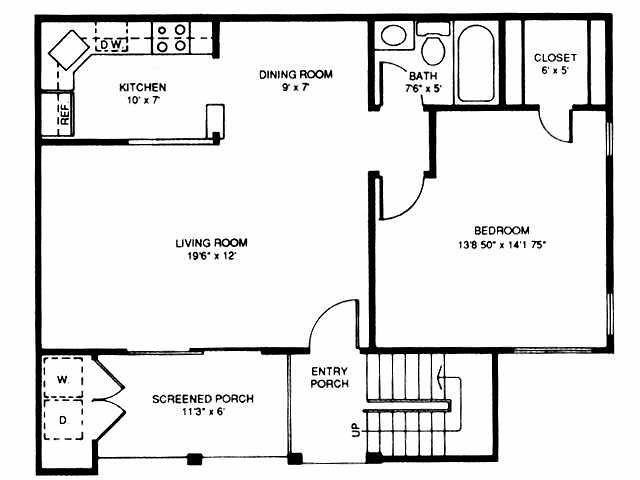This detailed floor plan of a house features various well-defined living spaces. At the top left, there is a kitchen measuring 10 feet by 7 feet, equipped with a refrigerator, corner sink, dishwasher, and stove. The kitchen flows seamlessly into a dining room that measures 9 feet by 7 feet through a connecting doorway. Below the kitchen and dining room is a spacious living room, measuring 9 feet 6 inches by 12 feet.

To the right of the kitchen is a bathroom measuring 7 feet 6 inches by 5 feet, complete with fixtures including a sink, toilet, and bathtub. Adjacent to the bathroom is a compact closet space measuring 6 feet by 5 feet. Below these spaces is a square-shaped bedroom, boasting generous dimensions of 13 feet 8 inches by 14 feet 1.75 inches.

The lower portion of the layout, beneath the living room and bedroom, includes a multifunctional area. It features a laundry space with a washer and dryer, a screened porch measuring 11 feet 3 inches by 6 feet, an entry porch area, and what appears to be a staircase for added accessibility.